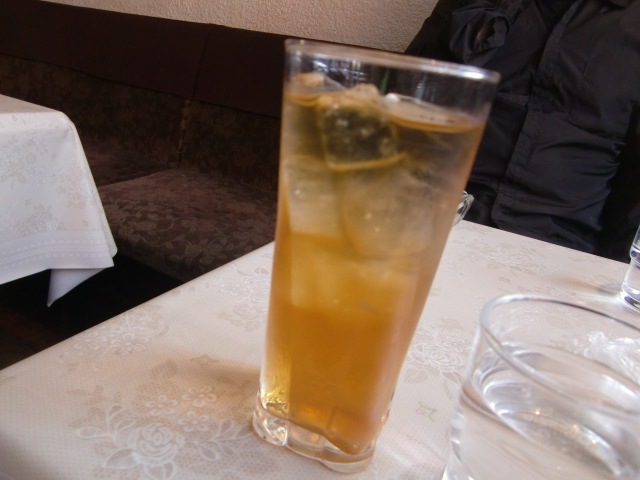In this detailed photograph taken in a sophisticated restaurant, the foreground is dominated by a dining table adorned with a white linen tablecloth featuring rose patterns. Two glasses of water are placed on the table, one barely visible and the other partially visible, along with a clear glass containing a light brown iced drink, possibly iced tea. The table, positioned on the right, occupies most of the frame, while a smaller table with a similar tablecloth is seen on the left. The background displays a cushioned, dark burgundy booth running along the wall, where a person in a dark shirt—possibly black or deep blue—is seated. This person is framed against a white wall, enhancing the contrast of the scene. The overall color palette includes shades of brown, black, white, and burgundy, adding to the restaurant's warm and inviting ambiance.